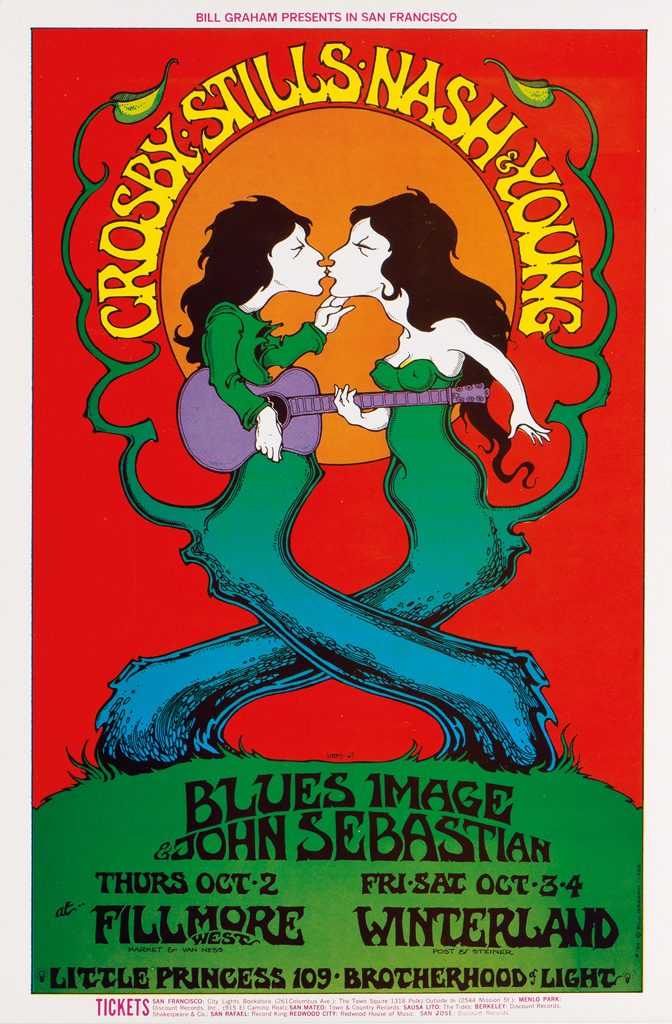This poster for a music festival presented by Bill Graham in San Francisco features a vivid, psychedelic design. At the top, in a white border with pink text, it announces "Bill Graham presents in San Francisco." Centrally, the names "Crosby, Stills, Nash, and Young" are displayed in yellow, hippie-style letters surrounding an image of two mermaid-like women with black hair and white skin, facing each other with puckered lips, almost kissing. The siren on the left holds a purple guitar. These mystical figures, with green and blue mermaid-styled outfits, appear to stand on lawn-like green grass. Below them, in black text over the green background, are details for performances by Blue's Image and John Sebastian on Thursday, October 2nd at Fillmore West, and on Friday and Saturday, October 3rd and 4th at Winterland. Further down, the poster lists acts Little Princess #109, Brotherhood, and Light. The background behind the women transitions from orange to red, and there’s a ticket information section in pink text at the bottom left, with multiple locations including San Francisco and San Mateo.